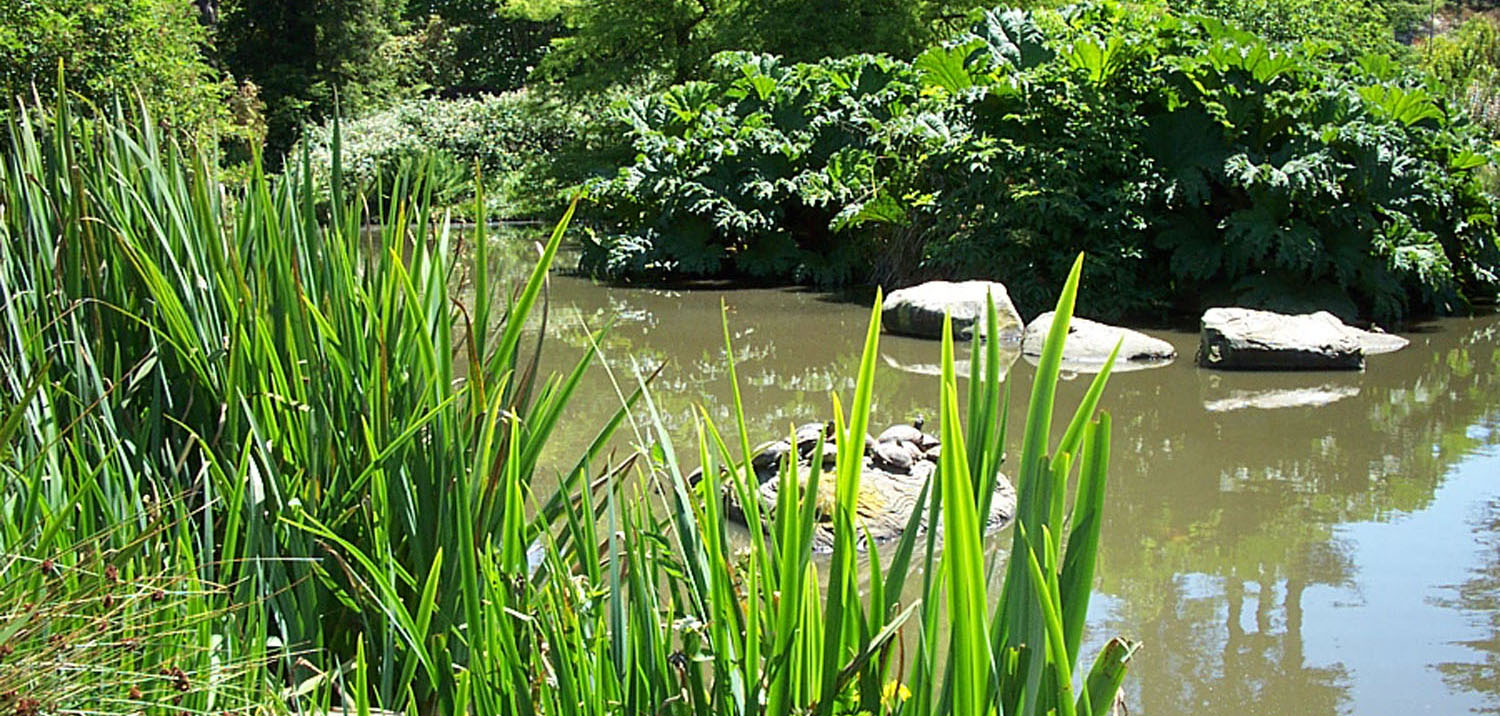The image depicts a serene natural scene with a creek or river featuring murky, brownish-green water. The area is adorned with lush greenery, including tall ferns and various shrubs whose leaves extend over the water on both sides. In the foreground, shoots of grass of varying lengths are visible. There are several boulders partially submerged in the water, with one prominent boulder hosting approximately ten turtles basking in the sunlight. The sunlight streams through the trees and bushes in the background, illuminating the scene and highlighting the peaceful ambiance. This picturesque setting evokes the tranquility of a park or possibly an expansive private garden.